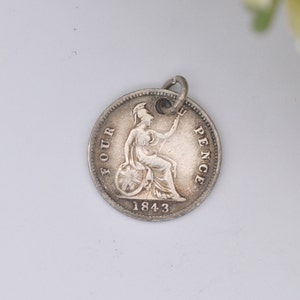This photograph showcases a Victorian-era silver 4 pence coin from 1843, intricately pierced and fitted with a chain-link ring, possibly for use as a necklace or keychain. The coin's weathered edges reveal a dark gray patina, contrasting with its polished center that highlights a detailed image. Engraved on either side of the central motif are the words "4 pence," with the date "1843" etched at the bottom. The central figure, distinct in Roman attire, is a stoic centurion or similar warrior, adorned with a traditional helmet bearing a Mohawk-like crest. The warrior, draped in a robe, appears seated on a shield or vessel, while raising a trident in one hand. The background of the image is predominantly gray, but a blurry, greenish object protrudes into the frame at the top right corner, suggesting the presence of a plant out of focus.